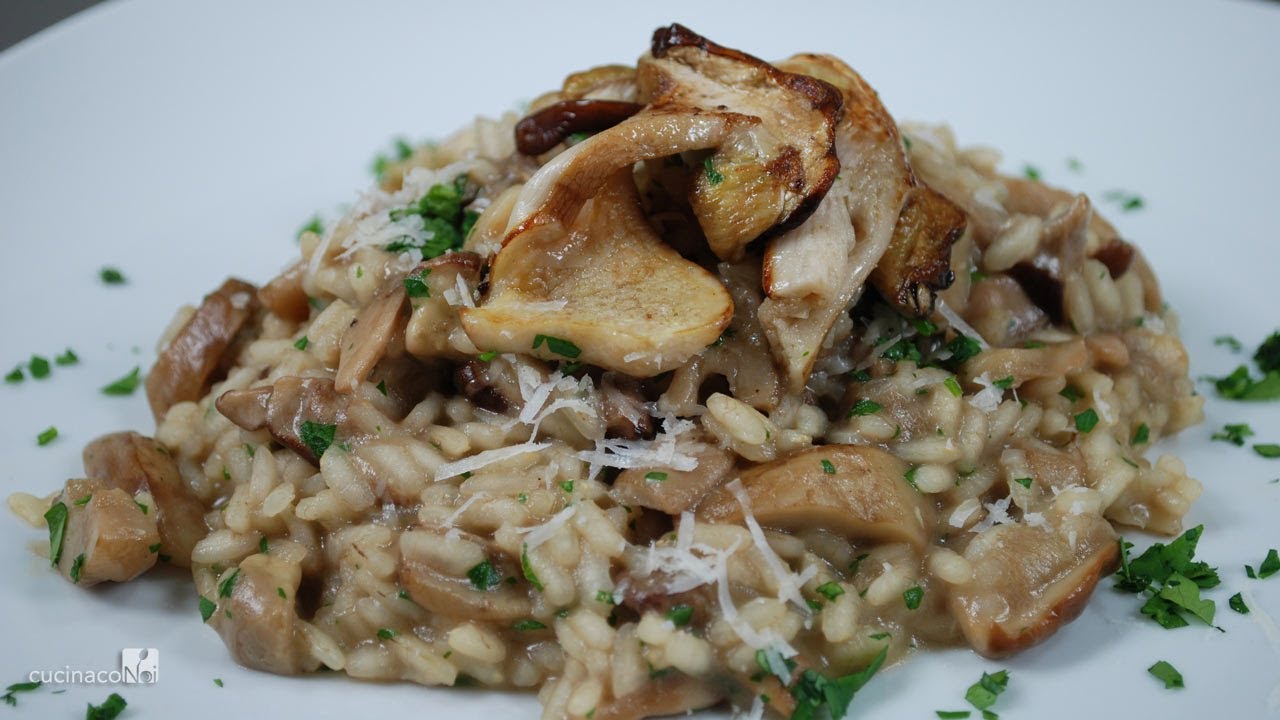On a large white plate, occupying almost the entire field of view, there lies a small, rounded mound of food, likely a mushroom risotto. The risotto comprises short-grain rice, forming a semi-cohesive mass, generously mixed with fried mushrooms. It features a number of brown, probably sautéed or fried mushrooms, that add texture and depth. Scattered throughout and on top of this heap are flecks of a green herb, most probably parsley, providing a splash of color against the otherwise brown and white palette. Additionally, there are hints of light-colored shreds along the mound, suggestive of shredded cheese. The pile of food, roughly the size of a hand, appears to be meticulously plated, with some pieces of chicken adding layers of both white and dark hues, possibly having some char marks for added visual and flavor dimensions. This carefully garnished dish looks both visually appealing and appetizing.